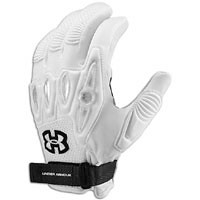The image features a detailed, high-contrast photograph of a white sports glove, prominently branded with the Under Armour logo on the wrist strap. The glove, showcased against a plain white backdrop, exudes a futuristic aesthetic with distinct design elements. The back of the glove reveals the thumb, forefinger, middle finger, ring finger, and part of the pinky finger. The fingers are articulated with accordion-style joints, making them flexible and padded, ideal for gripping. The black Velcro fastener secures the glove at the wrist, complemented by a black band featuring the Under Armour label. The glove also displays a complex pattern of circles, triangles, and horizontal stripes across the knuckles, adding to its technical appearance. This versatile glove seems suitable for various activities, possibly ranging from dirt biking or motorcycling to snowboarding or skiing, providing both protection and dexterity.